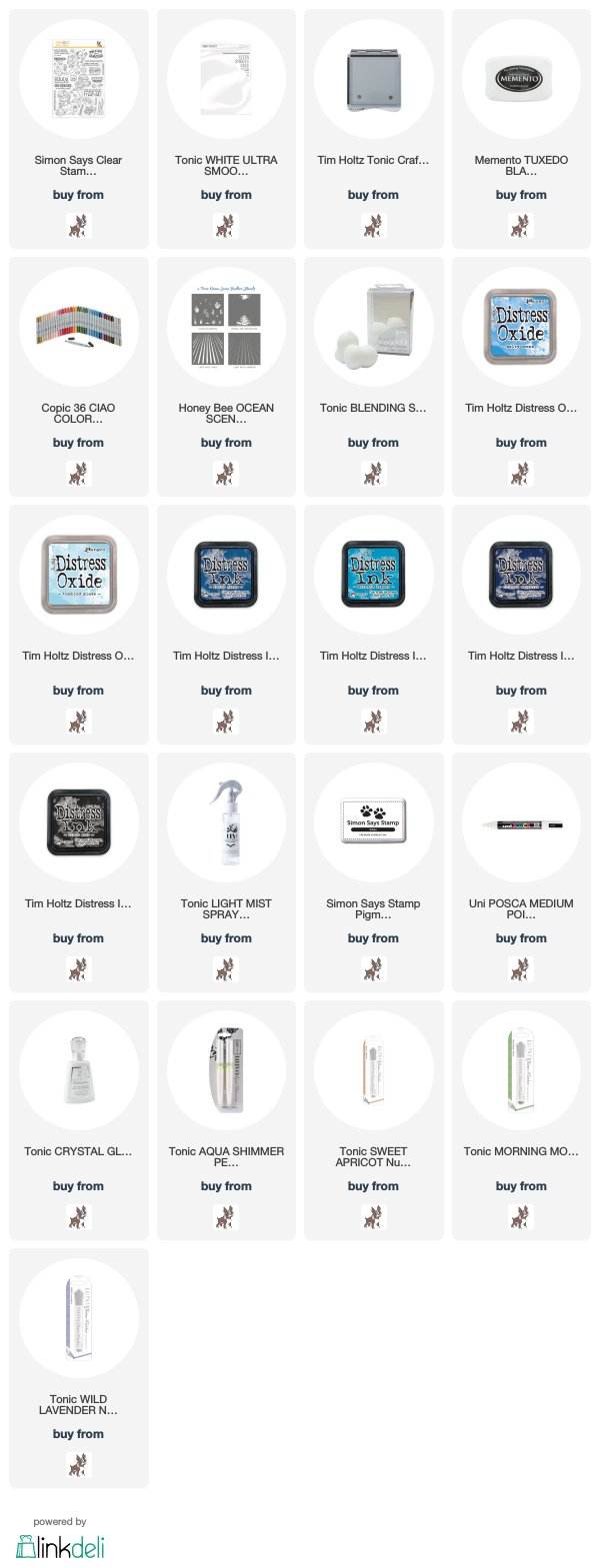This image is a screenshot displaying a selection of various supplies, organized in a grid layout. The grid consists of five rows with four items each, topped by an additional row featuring a single, left-aligned item. Each item in this arrangement is represented by a gray vertical rectangle housing a white, sideways oval, within which lies the object of interest. Below each object is a brief description of the item, followed by the phrase "Buy from" and a small image of an animated bulldog.

The available options listed beneath each description include:

1. Simon Says Clear Stamp
2. Tonic White Ultra Smooth
3. Tim Holtz's Tonic Craft
4. Memento Tuxedo Black
5. Copic 36-Ciao Colored
6. Honey Bee Ocean Scents
7. Tonic Blending Solution
8. Tim Holtz's Distress Oxide
9. Tim Holtz's Distress Ink (repeated several times)
10. Tonic White Liquid Mist Spray
11. Simon Says Stamp Pigment
12. Uni Posca Medium Point
13. Tonic Crystal Gloss
14. Tonic Aqua Shimmer
15. Tonic Sweet Apricot Nuvo

The screenshot provides a comprehensive view of the selection, featuring detailed graphics and concise item descriptions to guide potential purchasers.